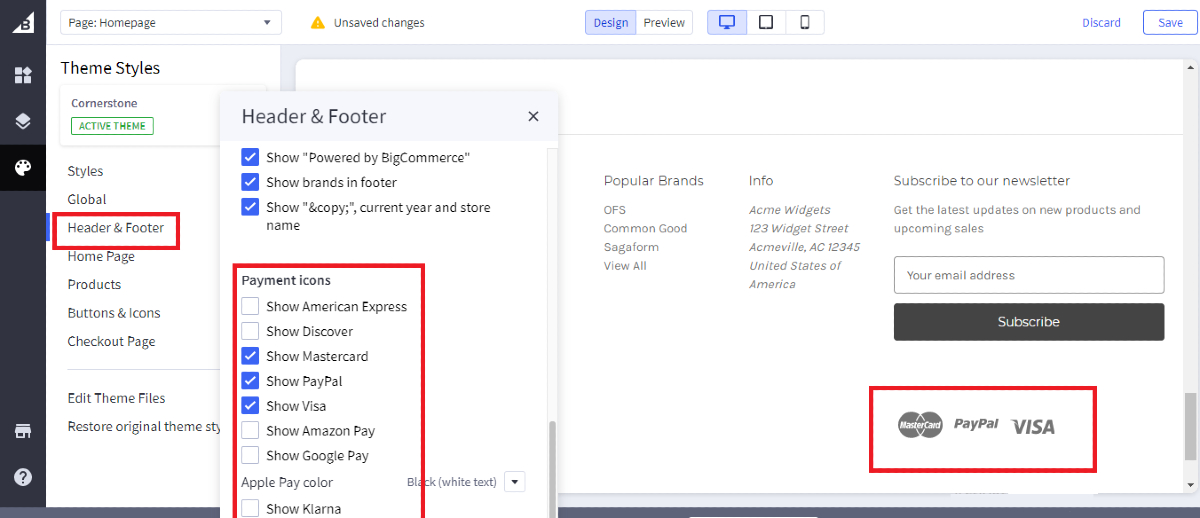The screenshot captures a web development interface displaying a page in design mode. On the left-hand side, there's a vertical sidebar with six white icons on a black background, each symbolizing different functions. The currently selected icon resembles a paint palette, while another is a standard help icon consisting of a circle with a question mark.

The top section of the interface outlines the current page, labeled "Home Page," and indicates that there are unsaved changes. Users can switch between "Design" and "Preview" modes and view how the page will look on different devices: a monitor, tablet, or cell phone, with the monitor view currently selected. To the far right are buttons for discarding or saving changes.

Within the sidebar, several menu items are listed, with "Header & Footer" highlighted by a red square, suggesting it's a screenshot rather than an active web page. Other menu items include "Theme Styles," "Home Page," "Products," "Buttons and Icons," "Checkout Page," "Edit Theme Files," and "Restore Original Theme."

When "Header & Footer" is selected, a pop-up menu appears, showing various options all ticked, such as "Show Powered by BigCommerce," "Show Brands in Footer," and "Show & Copy Current Year." Below these, there are options for displaying payment icons, with MasterCard, PayPal, and Visa currently selected. The screenshot also includes a preview section, displaying how these settings will appear when published on the webpage.